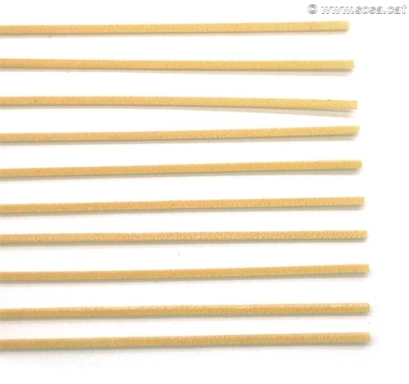The image depicts a set of long, skinny, beige-colored lines arranged horizontally on a pure white background, resembling fresh pasta noodles lightly dusted with flour. These lines, about ten to thirteen in number, are evenly spaced approximately an inch apart, and they all end at roughly the same length. Some of the lines have slight bends, adding a natural, imperfect appearance akin to authentic pasta. Shadows beneath each line enhance the texture, making the material somewhat ambiguous—it could be mistakably perceived as cardboard. In the top right corner of the image, there's a watermark featuring the letters "WWW" and "2021," alongside other partially legible characters like "OST," written in a small, gray font within a circle containing a "C."